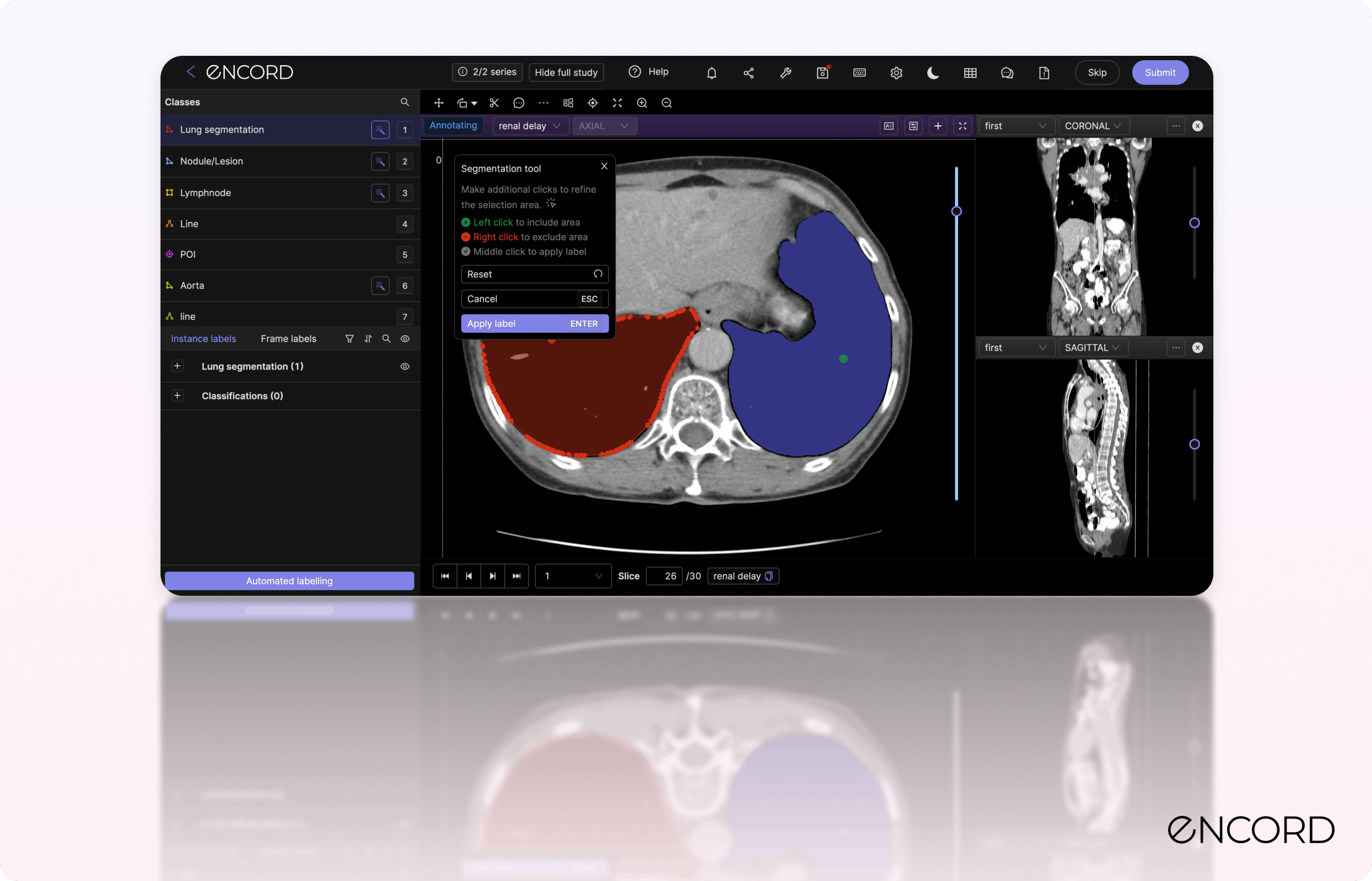The image depicts a black background with a computer screen displaying what appears to be medical imaging software named ENCORD, indicated by the text in the upper left and lower right corners. Dominating the center of the screen is a large, circular cross-section of possibly internal organs, featuring distinct red and blue areas which might signify different tissues or anomalies. Towards the left side of the screen, there is a column of small, unreadable text, while on the right side, there are two MRI-like images: one showing the spinal cord and the other illustrating the chest cavity, including the pelvis and hip area. Various menu options are visible on the far right, suggesting interactive elements for the software user. At the bottom of the central circular image, some indiscernible white markings add to the intricate details of the scan.